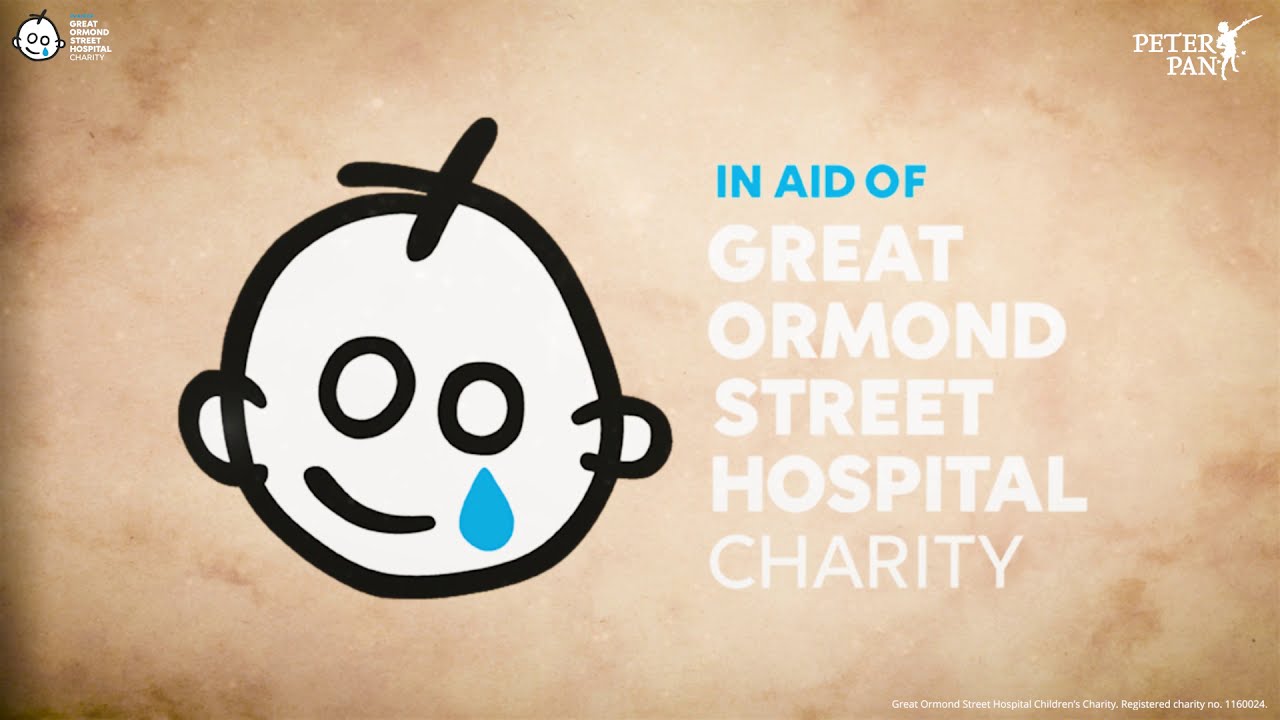The poster features a mottled beige background with dark patches, creating a textured appearance. On the left side, there's a simple, cartoonish face of a child, characterized by a thick black outline forming a circle for the head, with white circles for eyes and a small, curved line for a mouth, showing a smile. A prominent blue teardrop falls from one eye, and there are two black lines on the head representing hair, with ear shapes composed of a 'C' and a reverse 'C' on each side.

To the right of this face, large blue text in capital letters reads "IN AID OF," while below it, even larger white capital letters spell out "GREAT ORMOND STREET HOSPITAL CHILDREN'S CHARITY." The same child's face logo appears again in the upper left corner, alongside the text "Great Ormond Street Hospital Charity."

In the upper right, there's another logo featuring the silhouette of Peter Pan, a boy with his hand on his hip and pointing a sword upwards, next to the text "PETER PAN" in white capitals. Along the bottom right of the image, additional white text reads "Dark Registered Charity, number 1160024."